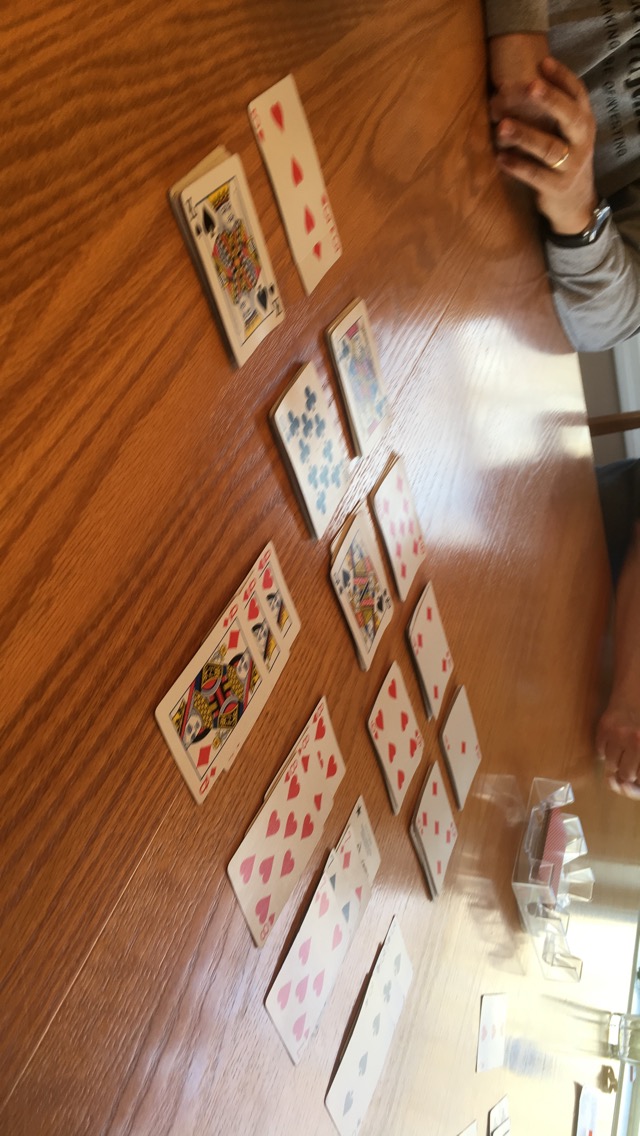A close-up photograph captures an elegantly designed, large light-colored table. The table features panel divisions, suggesting it can be extended for additional seating or functionality. Its highly reflective and shiny surface enhances the brightness of the room, accentuated by ample natural light streaming in from an open area at the rear of the photo.

On one side of the table, two people are seated with their arms visible. The man on the left wears a gold wedding band, a watch, and a long-sleeved gray shirt. Next to him, another man rests his folded hands on the table, indistinct except for his dark-colored shirt. In the center of the table, a plastic square holder contains a deck of playing cards.

A meticulous arrangement of playing cards is spread out across the table's surface. Prominently, three queens, one on top of the other, draw immediate attention. Nearby, stacks of the Eight of Hearts, sevens, and Three of Clubs are carefully organized, some laid out diagonally while others align horizontally across the table. The deliberate placement of cards and the serene tableau of the scene suggest an ongoing or recently concluded game, inviting viewers to ponder the narrative behind the image.